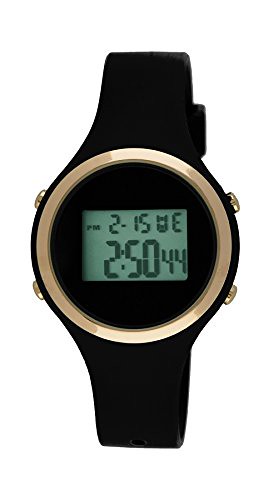This image showcases a modern digital watch against a white background, commonly found in online store catalogs. The watch features a thick black rubber strap and a striking brassy gold circular rim that frames the digital display. Four gold buttons are strategically placed around the watch face, positioned at the top left, bottom left, top right, and bottom right.

The central digital display is rectangular and relatively small, set within the round face of the watch. The main screen features the time, prominently showing 2:50 PM, with "PM" displayed in small print at the top. The display also shows the date, February 15th, alongside a day indicator, specifying Wednesday. Additionally, there is a smaller symbol that resembles a "U" followed by an "E," likely indicating battery life or another function. To the right of the main time, smaller digits "44" are visible, likely representing seconds. The simpler LCD technology of the display uses black numbers on a green background. The overall aesthetic of the watch combines traditional materials with a modern digital interface.